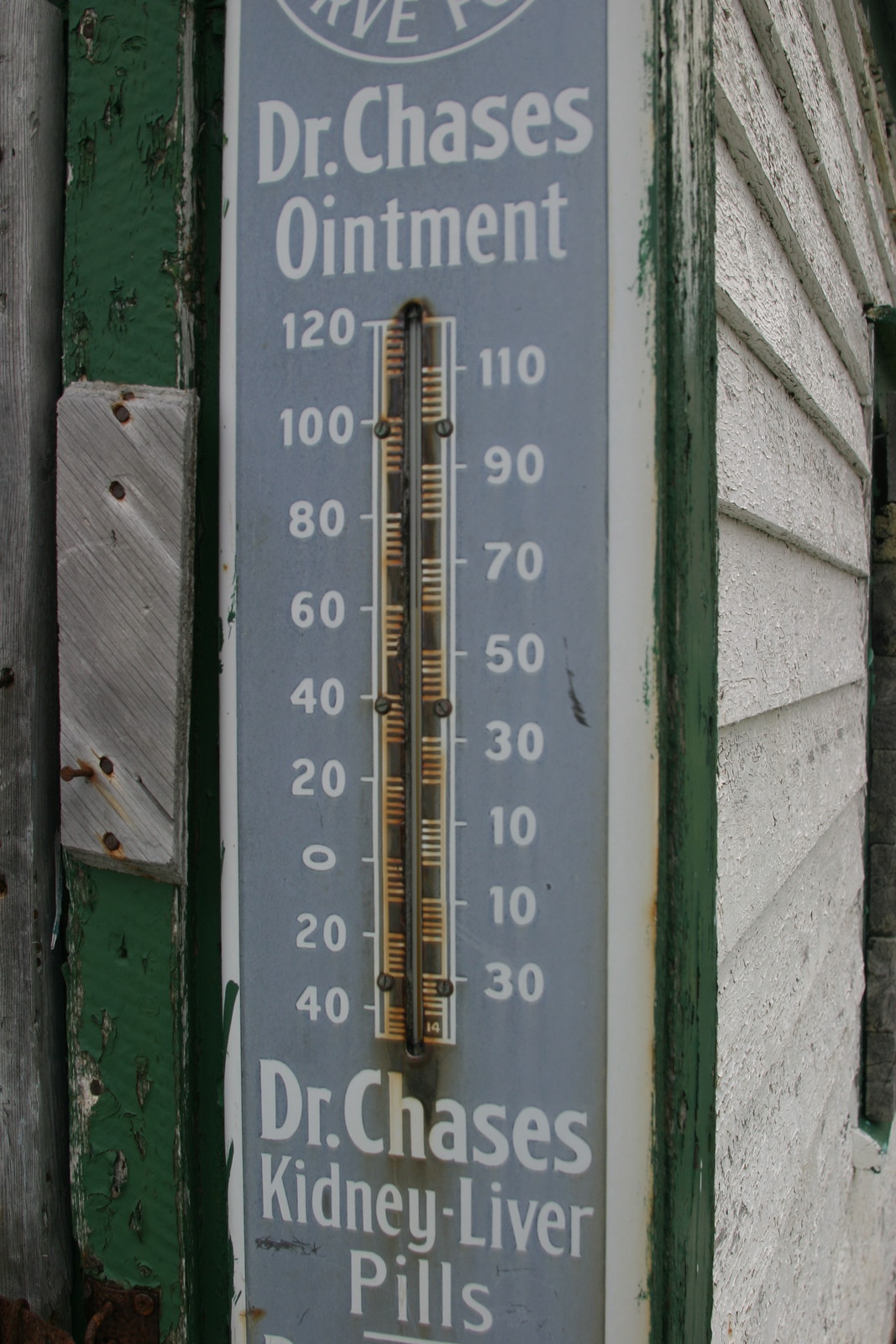An antique metal sign for Dr. Chase's Ointment and Dr. Chase's Kidney Liver Pills adorns the corner of a rustic building, right beside a door. The sign, which doubles as an old-school thermometer, is primarily a grayish-blue color with white text, though it appears heavily rusted, particularly around the thermometer component. The thermometer, now seemingly non-functional, features dual temperature scales, with Fahrenheit on the left ranging from 40 to 120 degrees and Celsius on the right ranging from 30 to 110 degrees.

The building itself adds to the nostalgic ambiance with its weathered white wood paneling and green accents, both showing significant signs of aging and wear, especially where the green paint has chipped away. The image captures a moment in time as a sliver of light from the right illuminates part of the building, enhancing the textured, timeworn feel of the scene, while the rest remains in shadow. There are no human elements present, allowing the viewer to focus solely on the historic and atmospheric details of the setting.